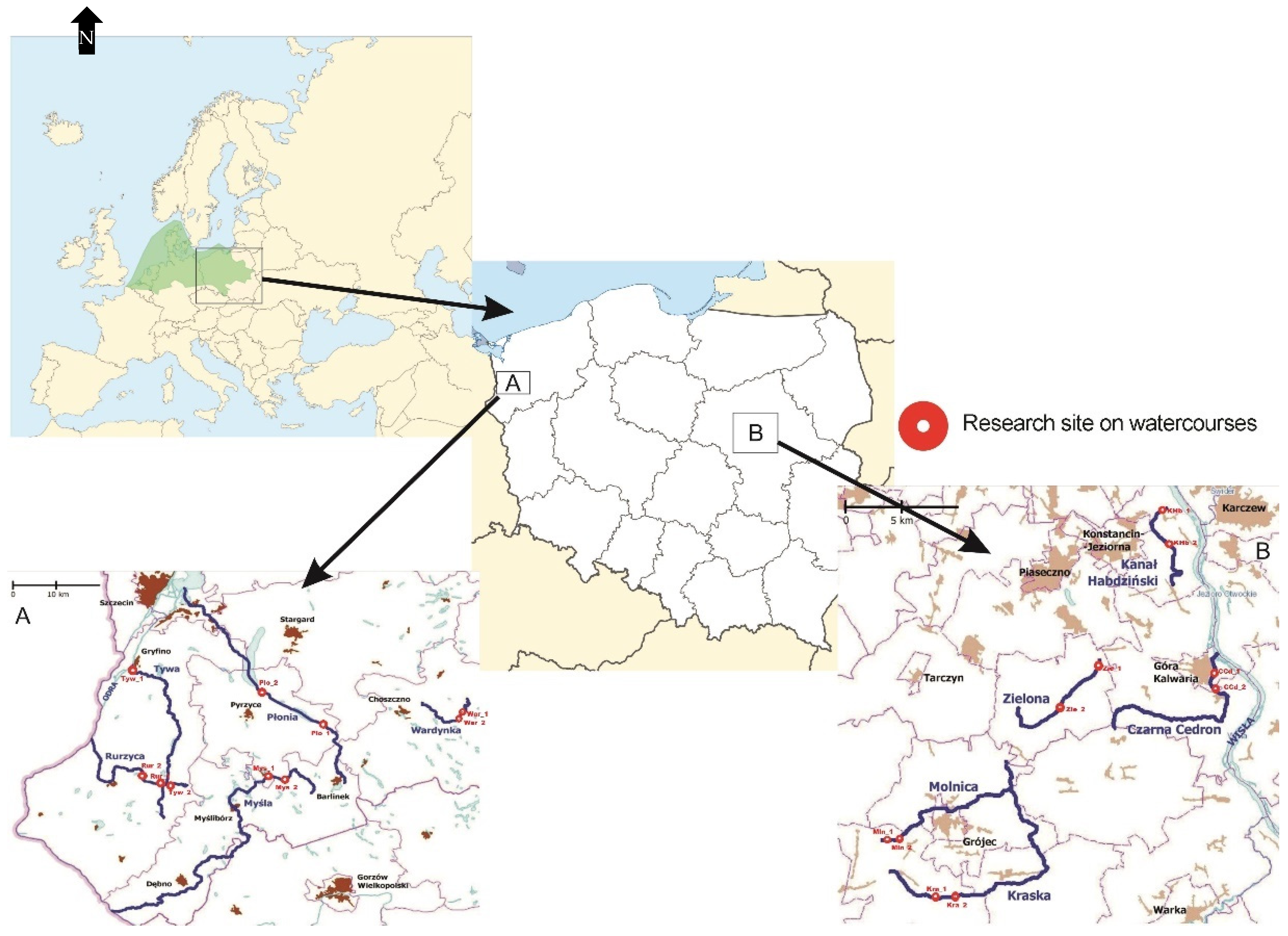This image features a set of four interconnected maps of a specific European country. The first map, located at the top left, highlights a region in green, with surrounding areas rendered in tan, and includes a northward arrow labeled "N" to indicate direction. Adjacent to this, another map displays the country in white, subdivided into various sections akin to counties. This map includes an "A" section marked on the top right, which directs to another closer regional map, while a "B" section points to yet another close-up map of the nation. Additionally, there is a distinctive circular icon resembling a target symbol, labeled "research site on water courses." Among the cities indicated on these maps are Monika, Grochek, Kraska, and Zelona, hinting at a Slavic or Russian influence. The layout of the maps suggests a detailed, step-by-step zoom-in of specific areas within the country, contributing to an overall intricate and layered cartographic presentation.